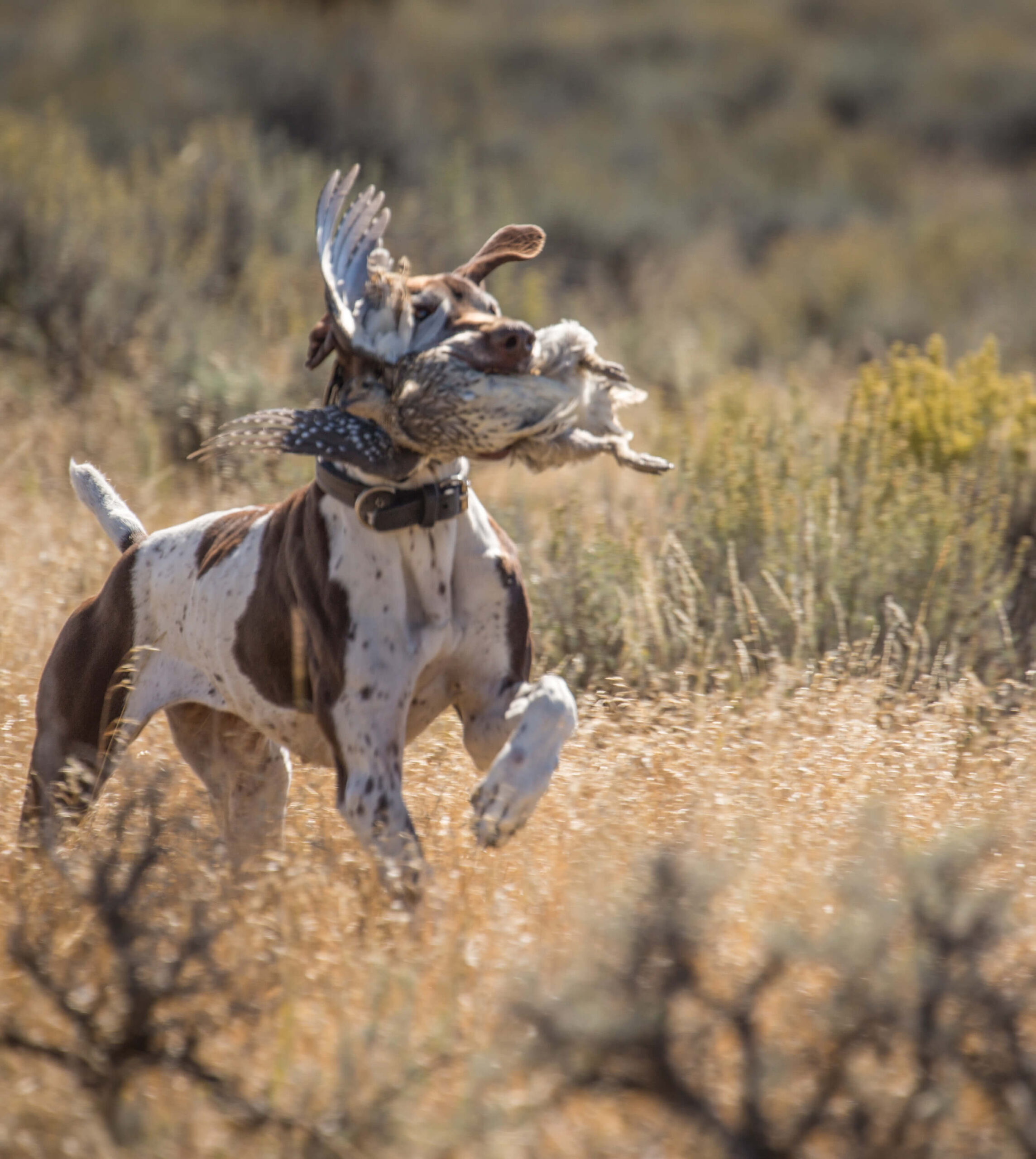In the sun-drenched expanse of a lightly vegetated field, a vivacious brown and white hunting dog is captured in mid-run, showcasing his prowess. His fur is dappled with white and brown spots, giving him a distinct and striking appearance. The dog, possibly a pointer breed, exhibits boundless energy as he gallops through the terrain with an unmistakable sense of pride. Clutched firmly in his mouth is a sizable bird, whose earthy brown and white feathers blend almost seamlessly with the dog's own coloring, though the full details of the bird are obscured. The bird is clearly lifeless, likely retrieved as part of a hunt. Adorning the dog's neck is a brown leather collar, complementing his athletic and focused demeanor. Surrounding them is a landscape painted in muted earth tones, with spindly, lifeless plants offering a stark contrast to the vibrant activity of the scene. Despite the sparse greenery, the bright sun casts a warm glow over the tableau, highlighting the dog's excitement and the thrill of the chase.